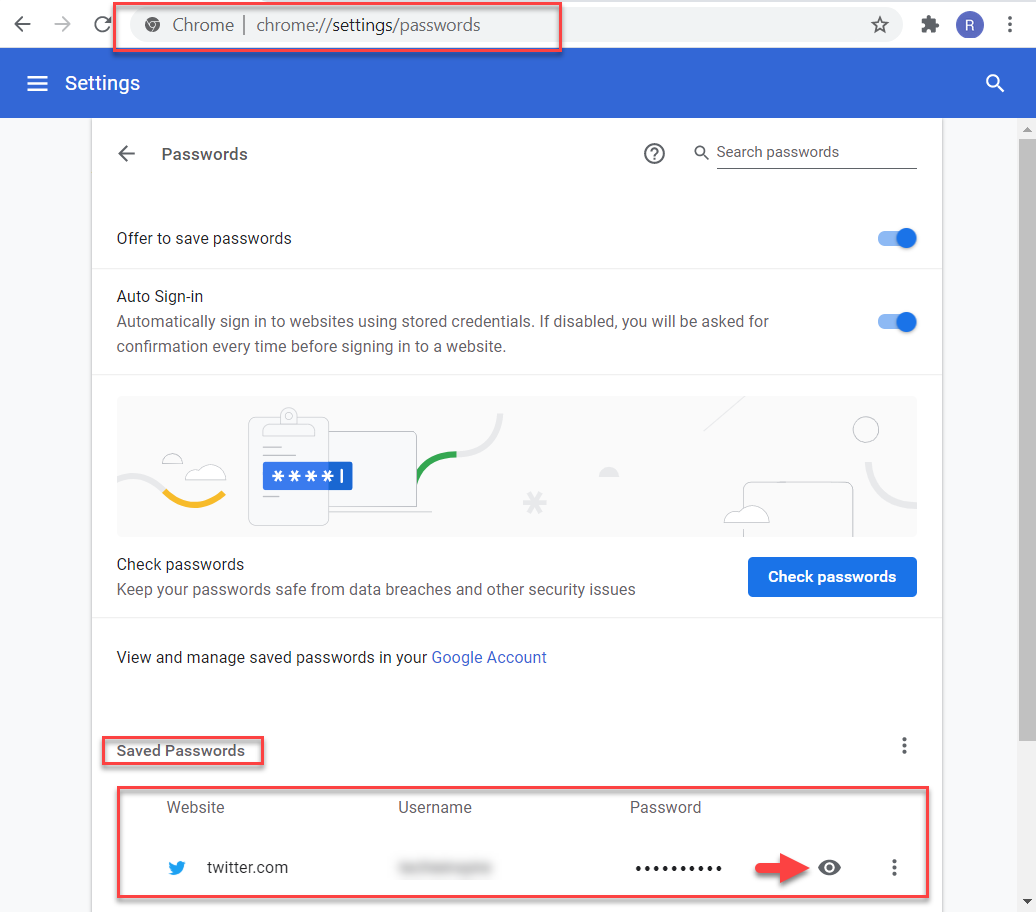The image depicts a Chrome browser window focused on the settings menu, specifically the passwords section. At the top of the window, there is a familiar toolbar that includes a backward and forward navigation button, a refresh button, and the Chrome logo. Within the address bar, it shows that the user is currently on the "chrome://settings/passwords" page. Adjacent to the address bar, there is a star icon for bookmarking, followed by a puzzle piece icon, a Rakuten emblem, and a three-dot menu icon for additional options.

Below the toolbar, a prominent blue rectangle spans the width of the page, featuring three horizontal bars signifying its function as a main menu. The word "Settings" is displayed in white text on this blue bar, and a small hourglass icon is located at the far end of it, indicating the presence of multiple search options within this settings page.

The page is aimed at allowing users to manage and protect their passwords, offering various tools and options to enhance password security. The overall layout is user-friendly but features an abundance of search interfaces within a small area, which may be perceived as excessive by some users.